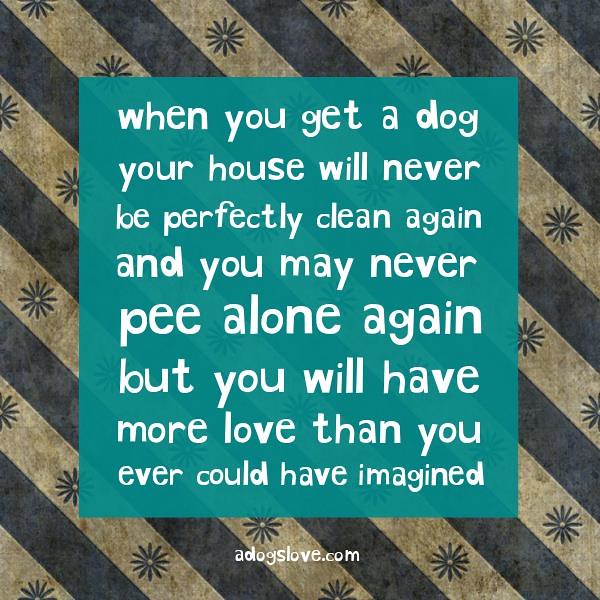This image features a whimsical and heartwarming macro with text on an opaque teal background. The text is written in playful white typography and reads: "When you get a dog, your house will never be perfectly clean again, and you may never pee alone again, but you will have more love than you could have ever imagined." The image is tagged with the website adogslove.com. The backdrop of the text features alternating white and gray vertical stripes adorned with starbursts on the white sections, adding a touch of charm. This playful and affectionate message is ideal for dog lovers and would make a meaningful gift, capturing the joy and love that come with owning a dog.